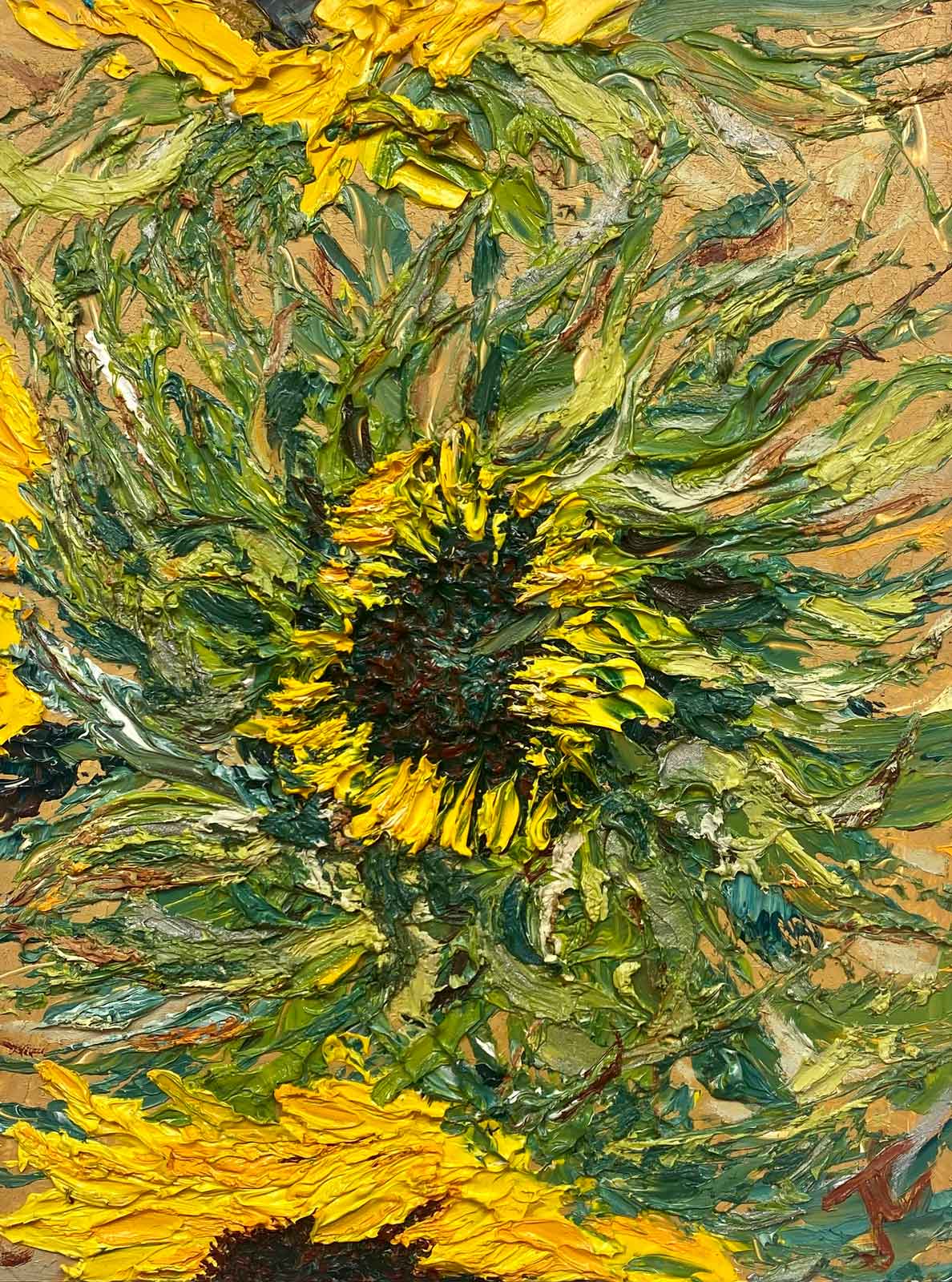This is a photograph of a dynamic, modern painting, executed in heavy oils or acrylics, portraying an abstract representation of sunflowers. The central focus is a large sunflower with radiant, thick yellow petals and a dark, intricately textured center in shades of brown, black, and green. From this central bloom, flowing, swirling green and blue leaves extend outward, creating a repetitive pattern across the canvas. The composition also includes partial views of additional sunflowers; one larger blossom peeks from the bottom left, and a section of another blossom is visible at the top. These supplementary sunflowers maintain the thick yellow petals and dark centers consistent with the central flower. All this is set against a pale, sandy-golden background that enhances the vibrant colors of the sunflowers. The portrait-style painting is signed "JC" in a distinct salmon pink signature at the bottom.